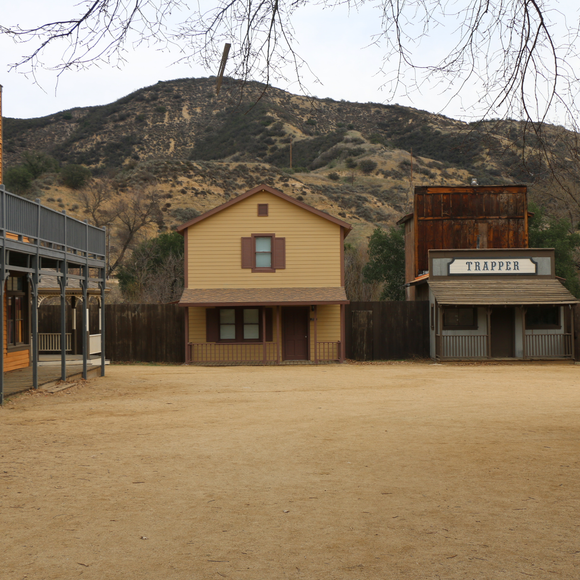This vertical image captures part of a meticulously maintained replica of an Old West town set against the rugged landscape of rolling hills covered in green and brown vegetation. A grayish sky looms overhead, with thin twigs hanging down from the top of the image, adding to the atmosphere. The focal point is a sandy, deserted town square flanked by three buildings. 

On the left, a beige two-story house with brown trim and shutters stands prominently. It features a dark brown roof, a balcony with a dark blue railing, supported by thin gray posts, and multiple windows framed in dark brown. 

Adjacent to it is a one-story light gray building labeled "Trapper" in gray letters against a white background. Behind this structure, a rusted building is partially visible, adding a sense of antiquity to the scene.

Further to the left, the edge of another two-story building is discernible, complete with a second-floor balcony and elegant gray railings and posts. The entire setting, devoid of people or animals, evokes a ghost town ambiance, enhanced by the dark wooden fence that separates the town from the lush hillside. The dusty, open foreground amplifies the sense of abandonment and timelessness.